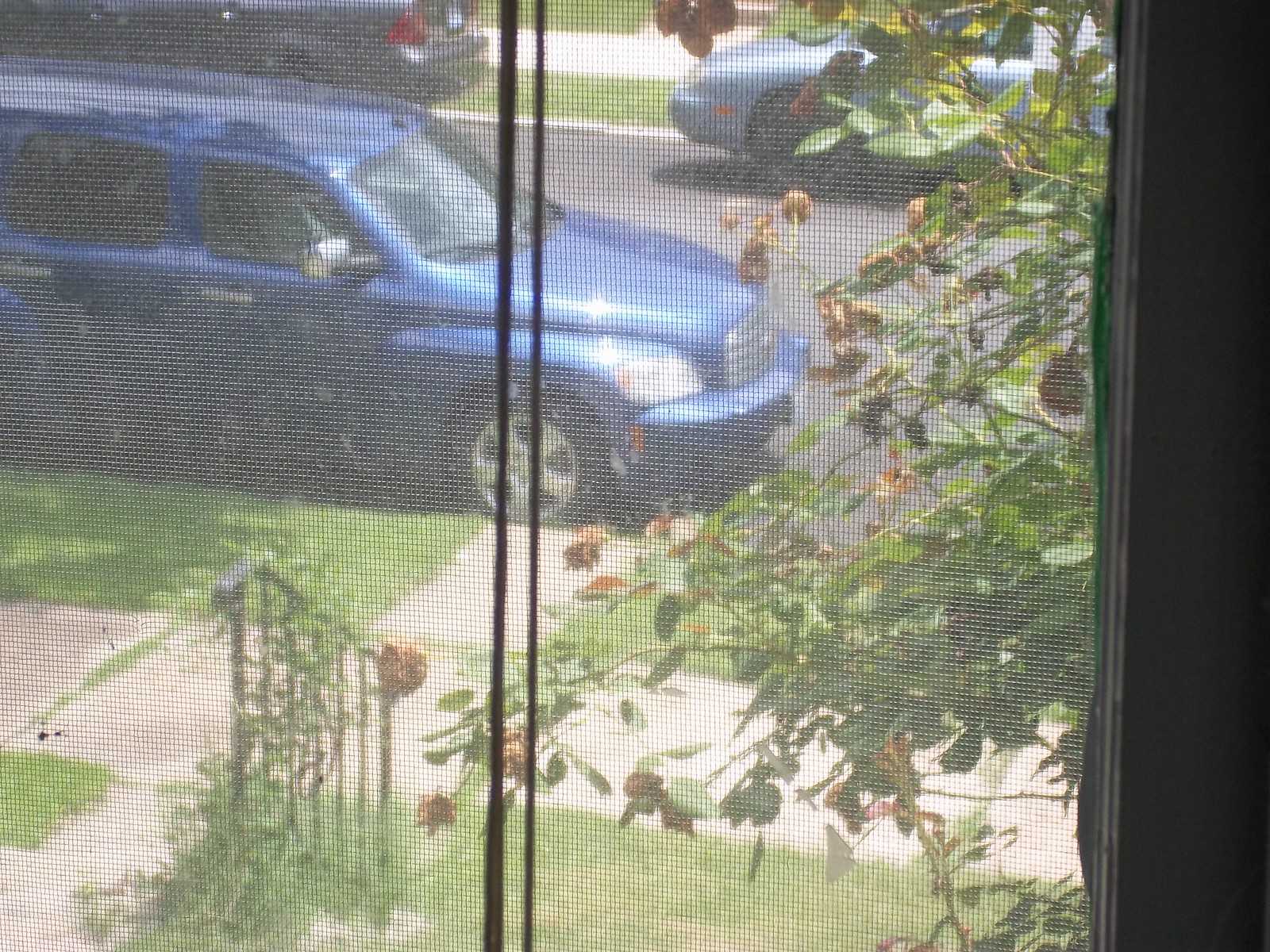A view from inside a house, looking out through a window screen, offers a peaceful suburban scene. In the foreground, the mesh of the screen creates a textured overlay. Just beyond, a tree or bush with green leaves partially obscures a well-kept lawn. The lawn extends to a tidy sidewalk, which then transitions to another patch of grass before reaching the street. On the street, a blue van is parked, with about three-quarters of it visible in the frame. Across the street, glimpses of two other cars can be seen, but only small portions are visible, hinting at more vehicles beyond the van. The overall scene captures a quiet neighborhood moment on a tranquil day.